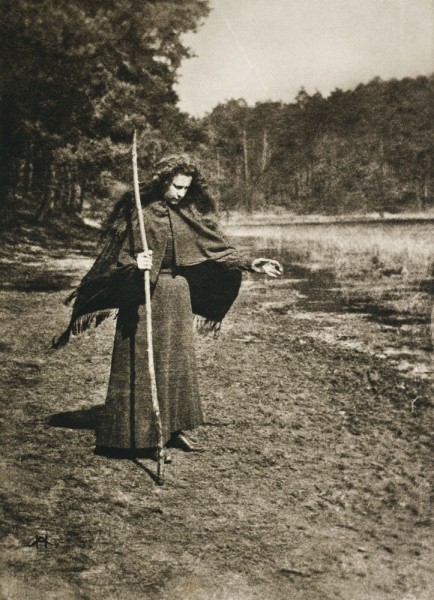This vintage black-and-white photograph captures a mysterious figure, seemingly a woman but with ambiguous facial features that suggest it could be a man. The individual is dressed in a long, dark floor-length dress made of rough fabric and a cloak-like shawl with tassels draped over their shoulders. Their dark, flowing hair cascades down past their shoulders. They hold a tall walking stick, or staff, in their right hand, which touches the ground and stands taller than them. Their left hand is extended outward and they gaze down towards the ground, evoking a sense of blessing or summoning.

The figure stands on a grassy and dirt-packed shoreline, adjacent to a body of water, possibly a stream or lake. Behind them, a densely wooded area creates a lush backdrop. The image, rendered in black and white with some almost sepia tones, evokes a striking, timeless ambiance.